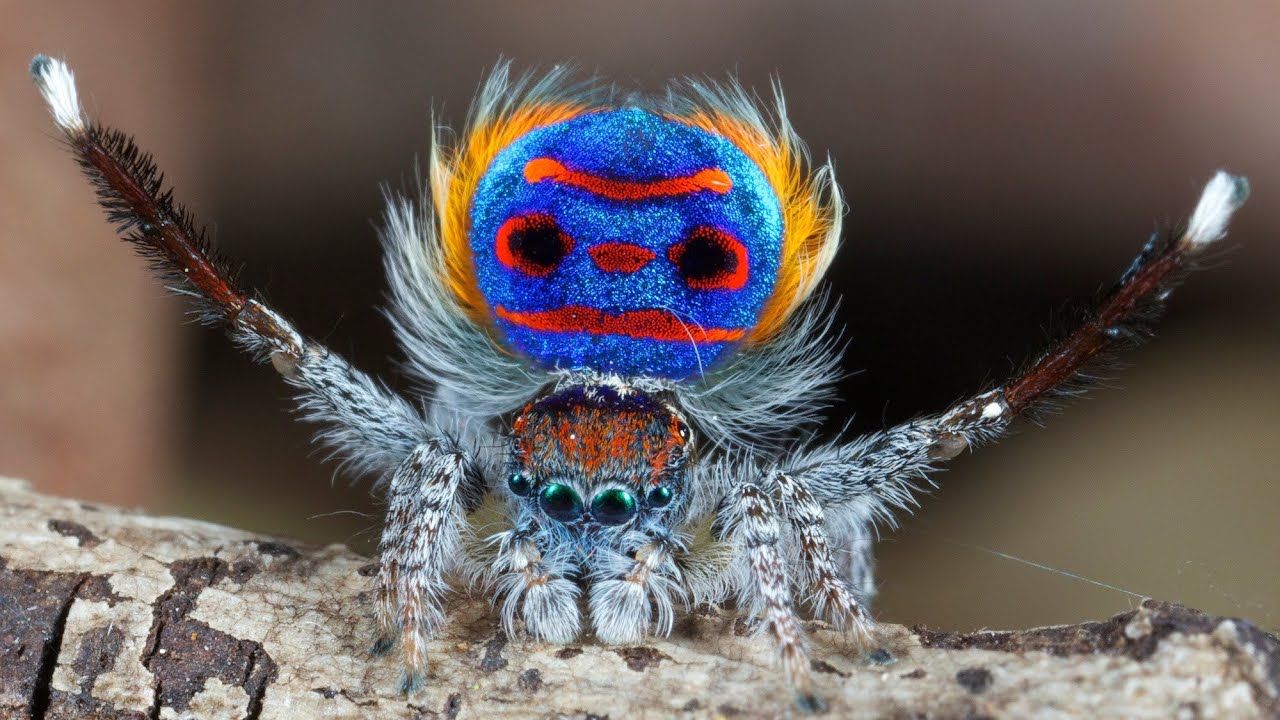In the image, there is a unique and intricately designed ornament resembling a spider. The spider has a round, blue head made of styrofoam with detailed facial features. It sports two red eyes with black pupils, a red nose, a red mouth, and a red line across its forehead. The head is surrounded by grey and orange fur on top and yellow and silver fur on the sides.

This captivating spider has two very long, spider-leg-like arms extending from each side, appearing to be composed of brown and white striped material akin to a bottle brush. Its body is adorned with four shiny, bright, dark green parts and is covered in luxurious fur that alternates between white and brown.

The spider ornament is positioned atop a dry branch, adding to its whimsical and lifelike appearance.